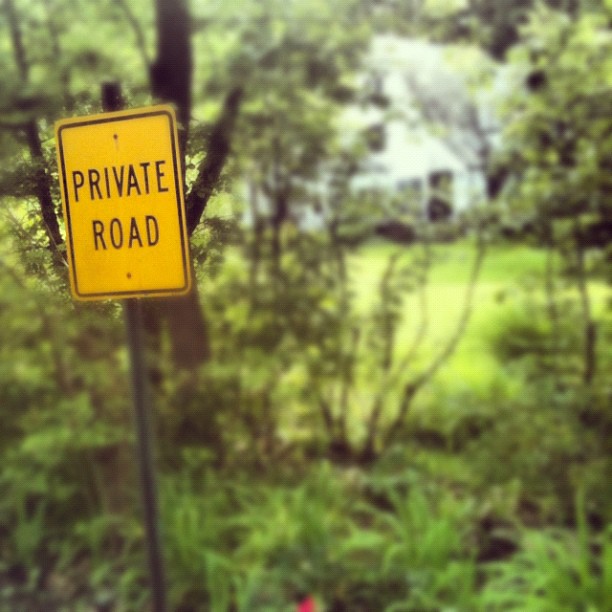In this photograph, a vivid yellow, vertically rectangular sign with a black border and the words "Private Road" in bold black text is centrally featured, mounted on a black metal pole anchored into the ground. The sign is the focal point, positioned in sharp clarity against a gently blurred backdrop of dense foliage and tall trees, with sparse branches allowing glimpses of a large, white house partially visible in the distance. The house, set amidst an expansive grassy yard and surrounded by greenery, has a hint of a window and perhaps a gray roofline. At the bottom of the photograph, a splash of yellow, likely a flower, adds an extra touch of color. The composition suggests that the private road indicated by the sign is a driveway leading up to the secluded white house.